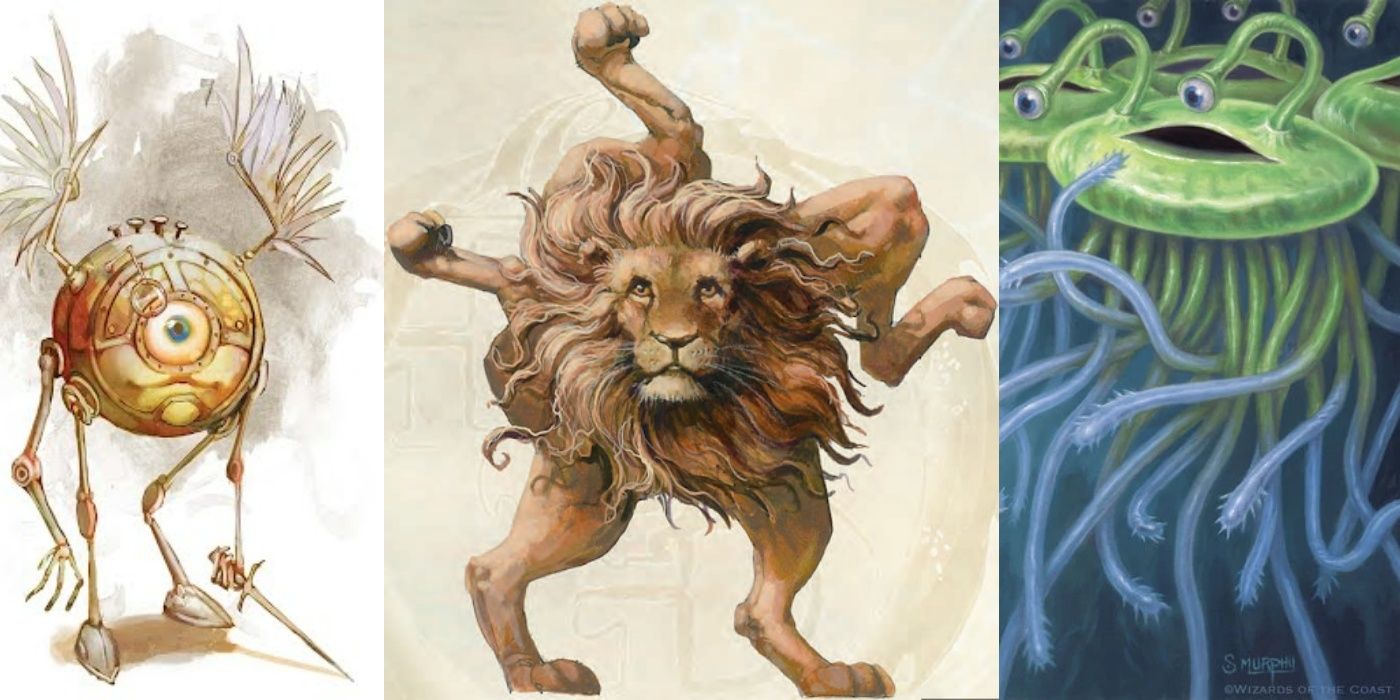The image consists of three drawings, arranged side by side from left to right, each depicting a fantastical creature. On the left, there's a gold stopwatch-like entity with an eyeball at its center, giving it the appearance of a Cyclops. This creature has legs, wings on its back, and two arms, one of which is holding a sword. The stopwatch character wears a forlorn expression. In the center, there's an unusual lion with five legs arranged in a dispersed manner across its body, almost forming a star pattern around its large mane, which gives it a radiant, sun-like appearance. The lion's face is serious and stern. On the right side of the image, a jellyfish-like creature floats, characterized by a large eye on the top of its bell and numerous green and blue tentacles hanging below. This jellyfish adds an extra touch of eeriness to the surreal assembly of creatures.